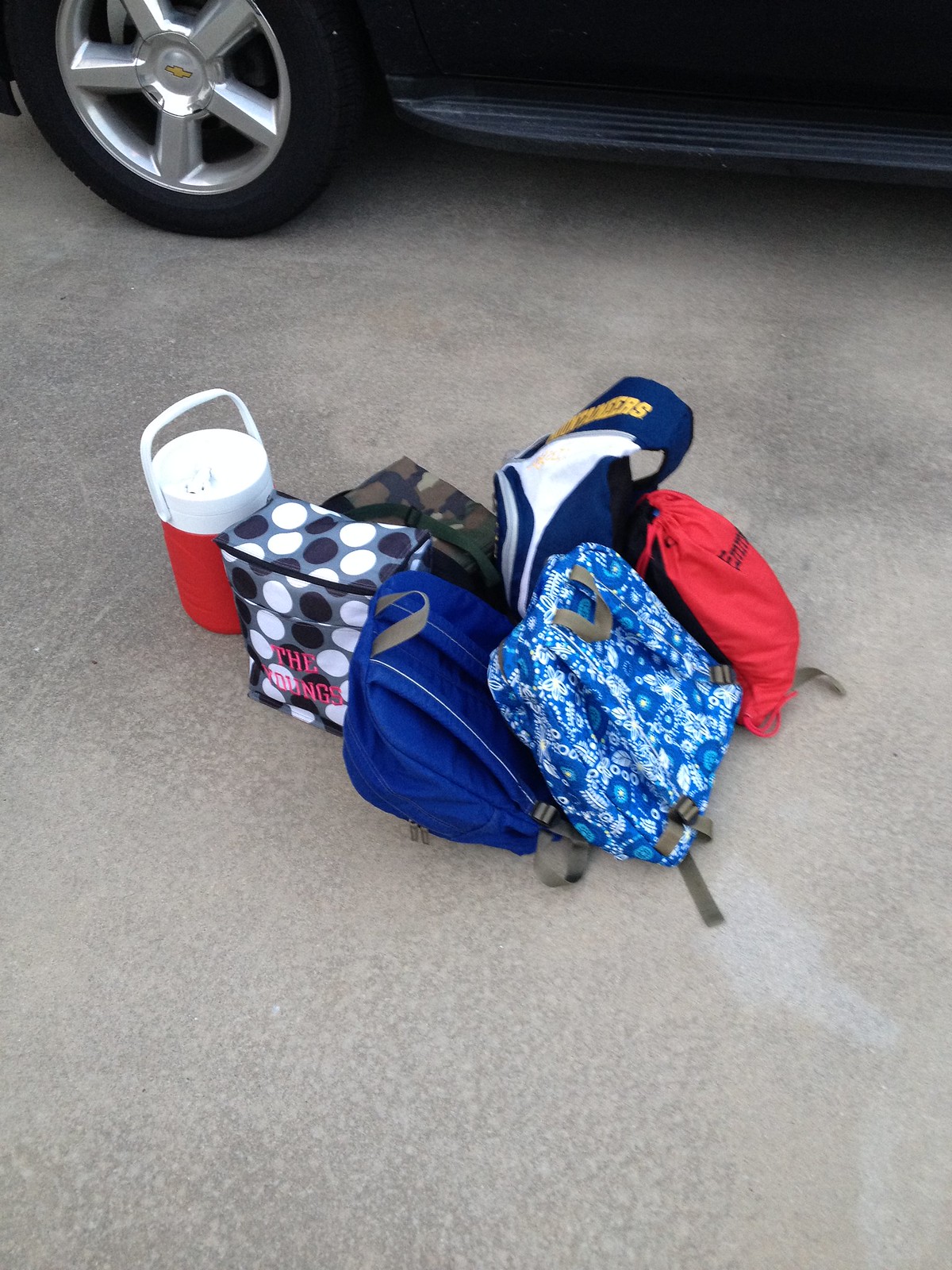The image captures an outdoor scene featuring various items placed on a concrete surface with the backdrop of a vehicle. From left to right, the top part of the photo is dominated by the side and running board of a Chevrolet car, identifiable by its emblem on a five-spoke chrome wheel and black tire visible at the bottom. Centered and spreading out across the image are several items laying on the asphalt.

Starting from the left-hand side, there's a red and white thermos with a pour spout, its handle upright. Next, a camouflage-patterned lunchbox is situated behind an oblong-shaped fabric container adorned with black and white circles and some indiscernible purple text. Moving clockwise, there's a dark blue and light blue backpack, followed by another blue and white backpack featuring yellow and white lettering that isn't legible.

Additionally, a red drawstring bag with unreadable text on it rests in the scene. The array of items concludes with a blue and white bag that is more rectangular, featuring backpack straps and a nylon webbing handle at the top. The overall composition highlights a juxtaposition of everyday carrying items against the mundane backdrop of a parking area.